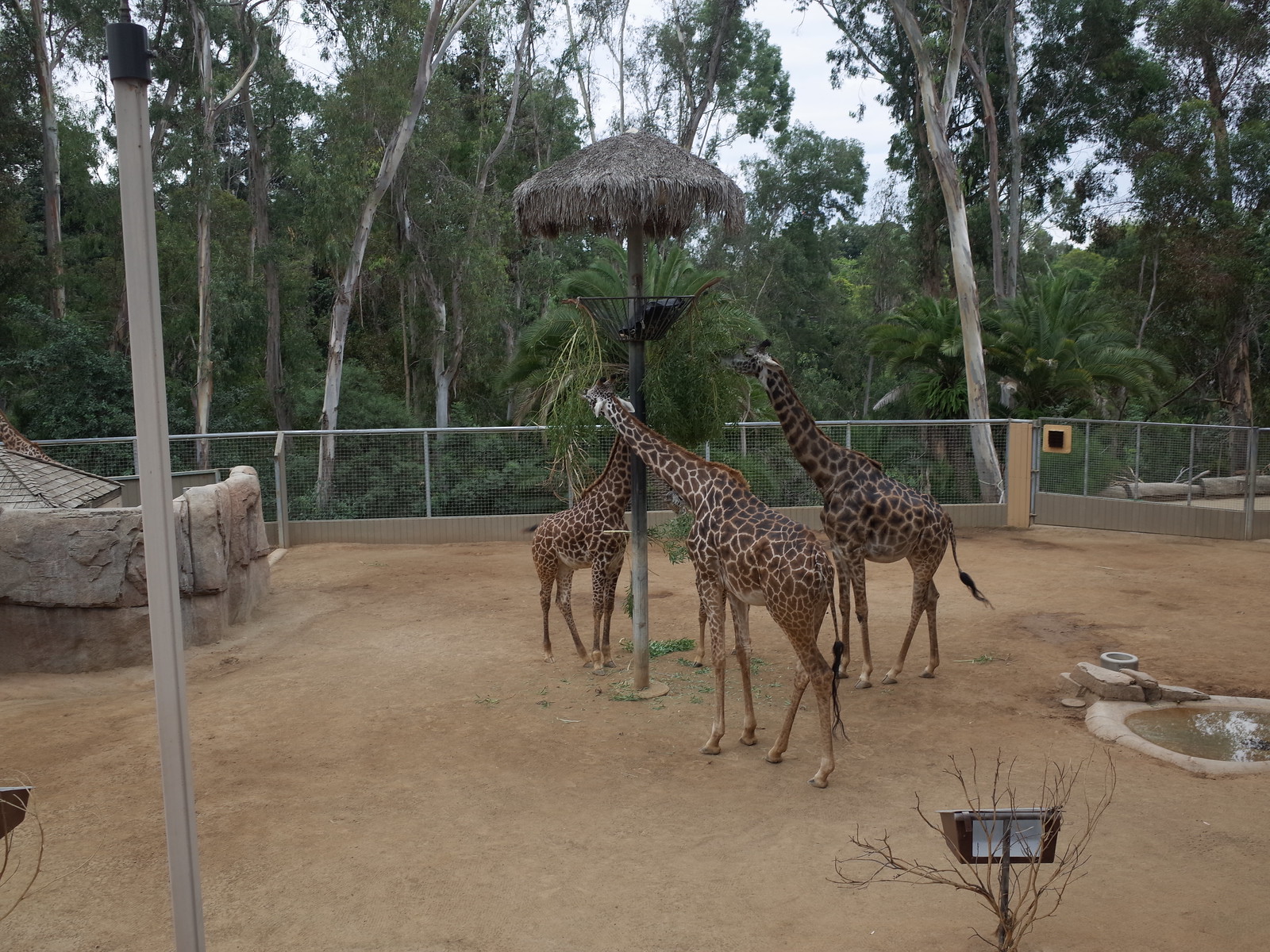The image depicts a color photograph taken outdoors, likely in a zoo or nature preserve. In the center of the image, three giraffes are sitting on a dirt-covered ground. They are close to each other and near a tall pole which features a container of grass and a thatched awning at the top, resembling a small hut, possibly providing shade. The giraffes appear to be getting water from a device at the base of this pole. Surrounding the enclosure are various elements including some rocks, a small pond filled with water to the right, and a light discreetly placed near a small tree to the left. The area is enclosed by a fence, and in the background, lush green trees with dense foliage can be seen. The setting hints at an environment designed to mimic African landscapes.